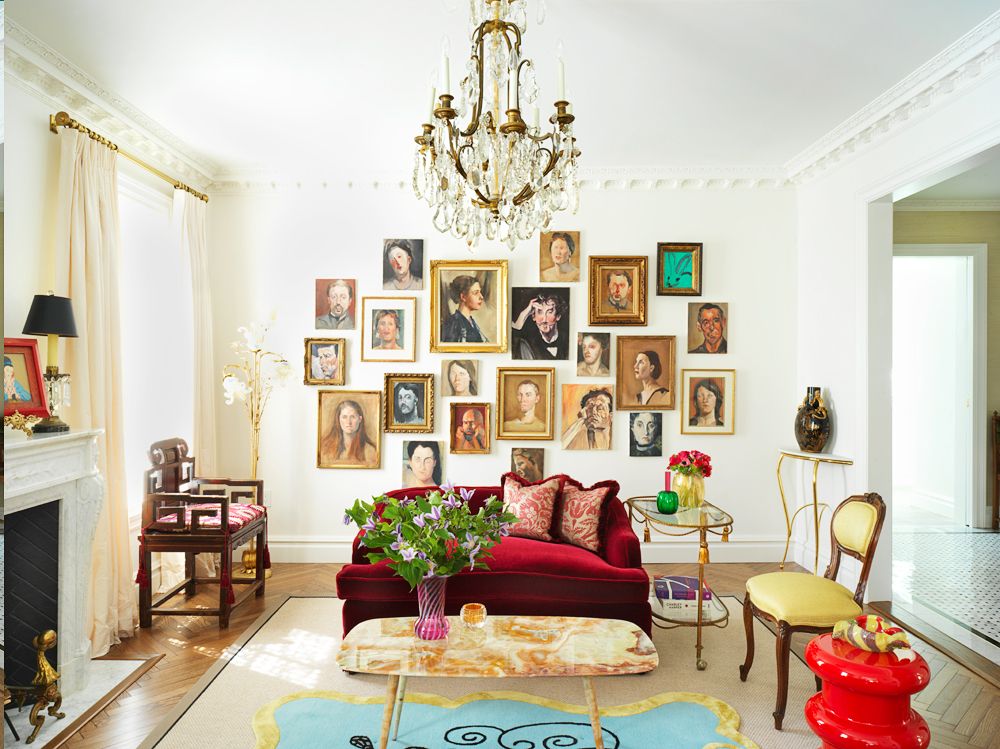This image depicts a detailed and vibrant living room with white walls and a warm, inviting atmosphere. The focal point of the room is a centered coffee table featuring a vase brimming with greenery and flowers, resting on a rug adorned with blue and yellow hues, with the yellow predominantly outlining the border. The elegant glass and gold chandelier hanging from the middle of the ceiling illuminates the room. 

At the back, a plush red sofa, accented with red-bordered throw pillows with red and white designs, sits against a wall. This wall is adorned with various hand-painted family portraits, each rendered in different artistic styles and mediums. To the right of the sofa, a glass end table holds another vase of flowers and assorted objects. A cream-colored chair with wooden legs is positioned nearby, with a small table and vase located behind it. Further right, a visible walkway leads to another room, suggesting a connection to the kitchen, hinted at by the tiled or marble flooring.

On the left side of the room, a white fireplace is topped with a lamp and a picture frame, providing a cozy touch. Adjacent to the fireplace, a single wooden chair with a seat cushion is placed near a window. This window, adorned with cream-colored curtains hanging from a brass rod, allows natural light to flood the room. The floor features a mix of wooden flooring and a secondary rug marked by black symbols. The overall decor, featuring wooden and upholstered furniture combined with intricate artistic accents, brings a sense of history and personality to the space.